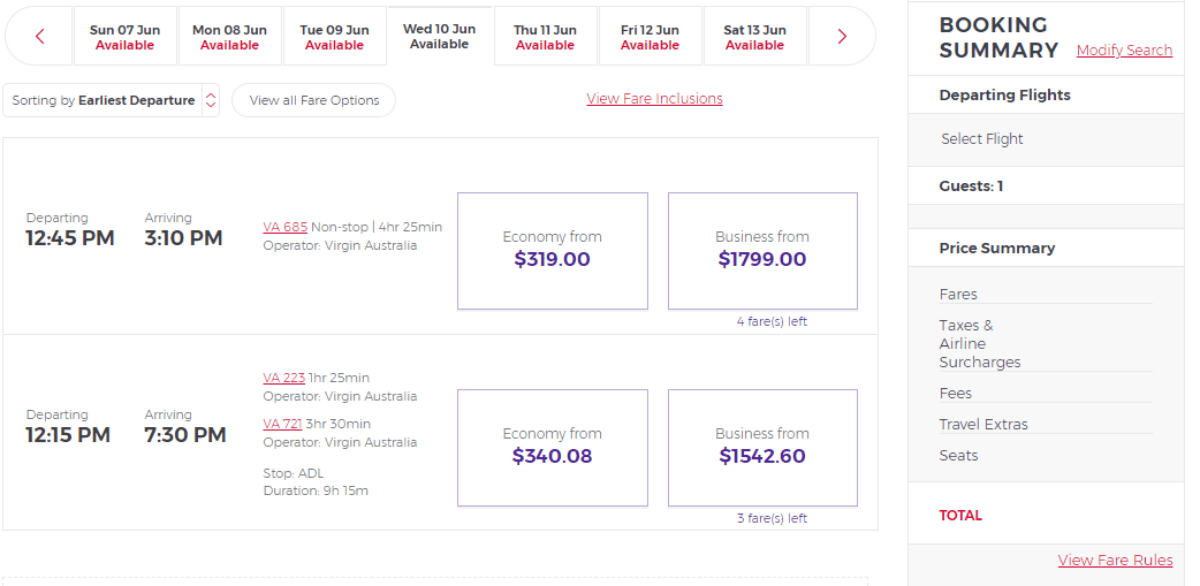The booking interface for a flight displays various tabs at the top, corresponding to different travel days. A left arrow appears before the dates, while a right arrow sits at the end. Seven dates are currently visible, starting from Sunday, June 7th, highlighted in black with "available" indicated in red beneath it. The subsequent dates include Monday, June 8th, Tuesday, June 9th, Wednesday, June 10th (currently viewed and also highlighted in black), Thursday, June 11th (marked as available in red), Friday, June 12th, and Saturday, June 13th.

Below these dates, on the far left, there's a sorting option labeled "Sorting by," with "Earliest departure" bolded and accompanied by a red up-down arrow. To the right, a bubble icon offers the option to "View all fare options."

Under the Friday section, there is an underlined red link titled "View fare inclusions." A box below displays departure and arrival details, split into two sections: the top section lists a flight departing at 12:45 PM and arriving at 3:10 PM, identified as VA 685, a non-stop flight lasting four hours. The economy fare starts at $319, while business class starts from $1799, with only four seats remaining. Another option shows a flight from 12:15 PM to 7:30 PM with multiple stop-offs, offering economy fares from $340 and business class from $1542.

On the far right, a vertical column contains a "Booking Summary" box, which includes options to "Modify Search," details of the departing flights, a pricing summary, and clickable "Fair Rules" for additional information.